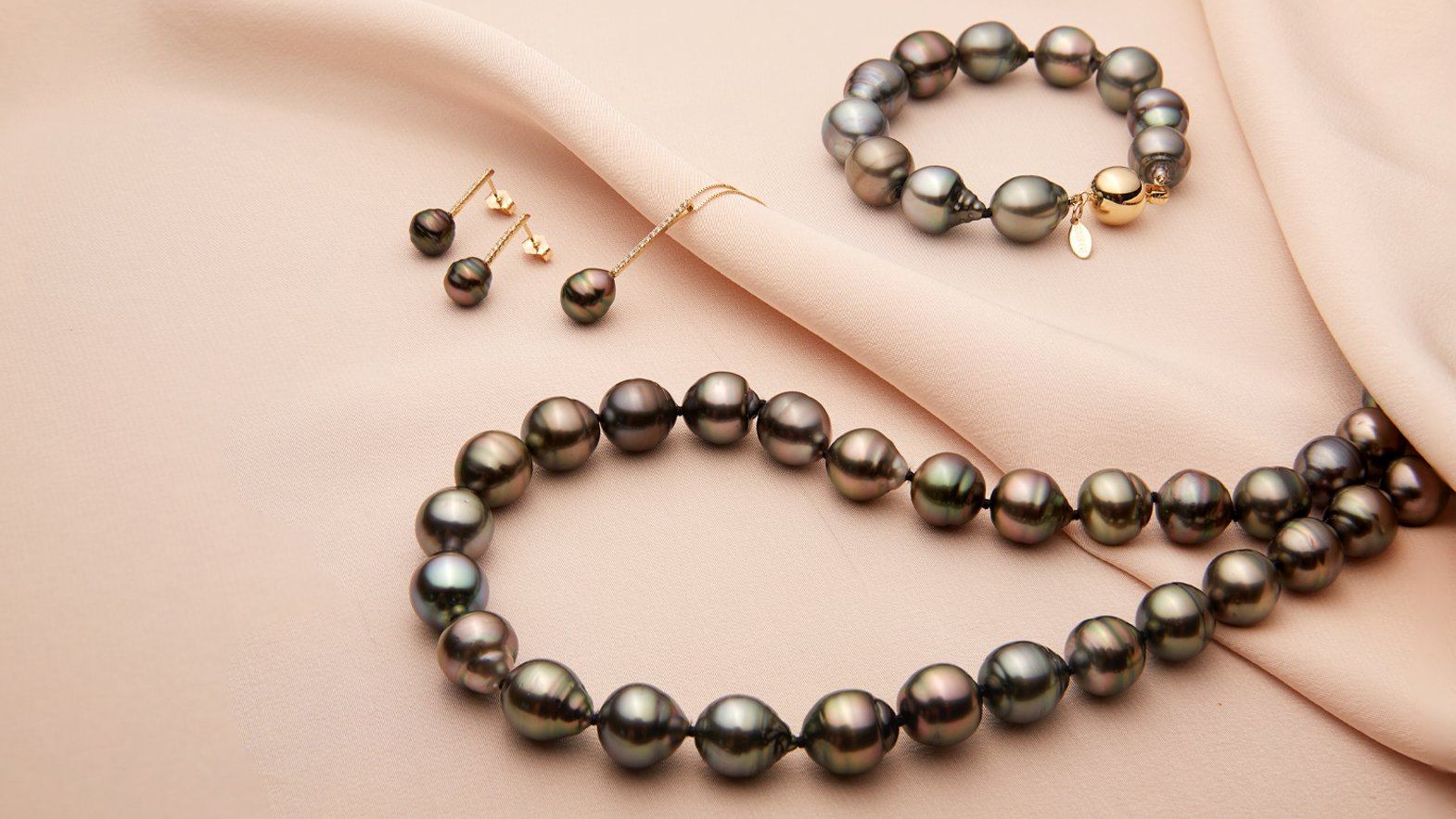The image showcases a collection of beaded jewelry artfully arranged on a pale, soft pink fabric background. The centerpiece is a striking beaded necklace composed of what appear to be dark, incandescent river pearls shimmering with shades of red, green, and blue. The necklace features slightly teardrop-shaped beads and extends across the fabric, partially hidden in the folds. Complementing the necklace is a matching bracelet, adorned with the same lustrous beads and secured by a delicate gold clasp, which adds an elegant touch. Additionally, there are a pair of matching earrings, each designed with a gold bar and small stones, as well as a single pearl pendant on a gold chain, featuring a similar gold bar design. The setup, characterized by its soft, bedroom-like quality, is perfect for a product image ideally suited for social media or a jewelry website.